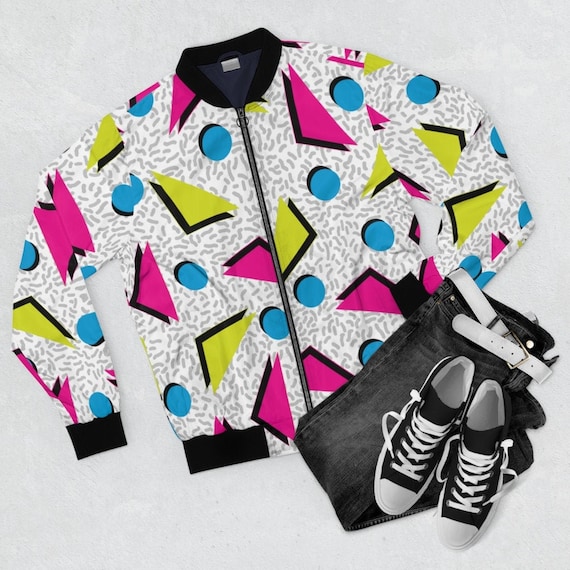This image features a meticulously arranged vintage outfit against a white background, capturing the essence of 90s fashion. The standout piece is a white jacket adorned with intricate patterns: gray, caterpillar-like squiggles serve as the backdrop, overlaid with neon pink and electric green triangles of varying sizes, all featuring black shadows for added depth. Blue circles, uniform in size and also with black shadows, are scattered across the jacket. The jacket boasts a black collar, black cuffed sleeves, and a black hemline, complete with a zip-up front. Accompanying the jacket, a folded pair of dark jeans—either deep blue or black—rests with a white belt threaded through its loops. Completing the ensemble, a pair of black and white Converse sneakers, characterized by their white laces and toes, are positioned at the bottom of the frame. This carefully curated outfit is displayed without a model, emphasizing the bold and nostalgic patterns and colors that define the era.